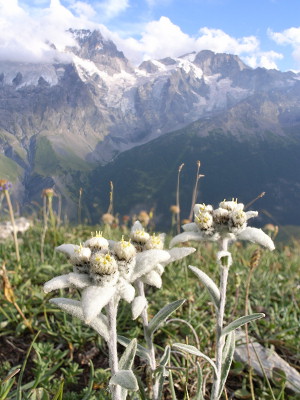In this daytime scene, we see a majestic mountain range, predominantly gray-brown with snow-capped peaks, set against a vibrant blue sky dotted with fluffy white and gray clouds. At the ground level, a green grass field abundant with various plants stretches out. In the foreground, a trio of distinctive white flowers with yellow stamens stand out. The flowers have fuzzy, minty-frost leaves and delicate white petals. Behind the flowers, the mountain's dark gray and green patches hint at more vegetation. The overall composition captures the serene beauty of the outdoors, blending rugged mountains with the delicate charm of wildflowers under a lightened sky.